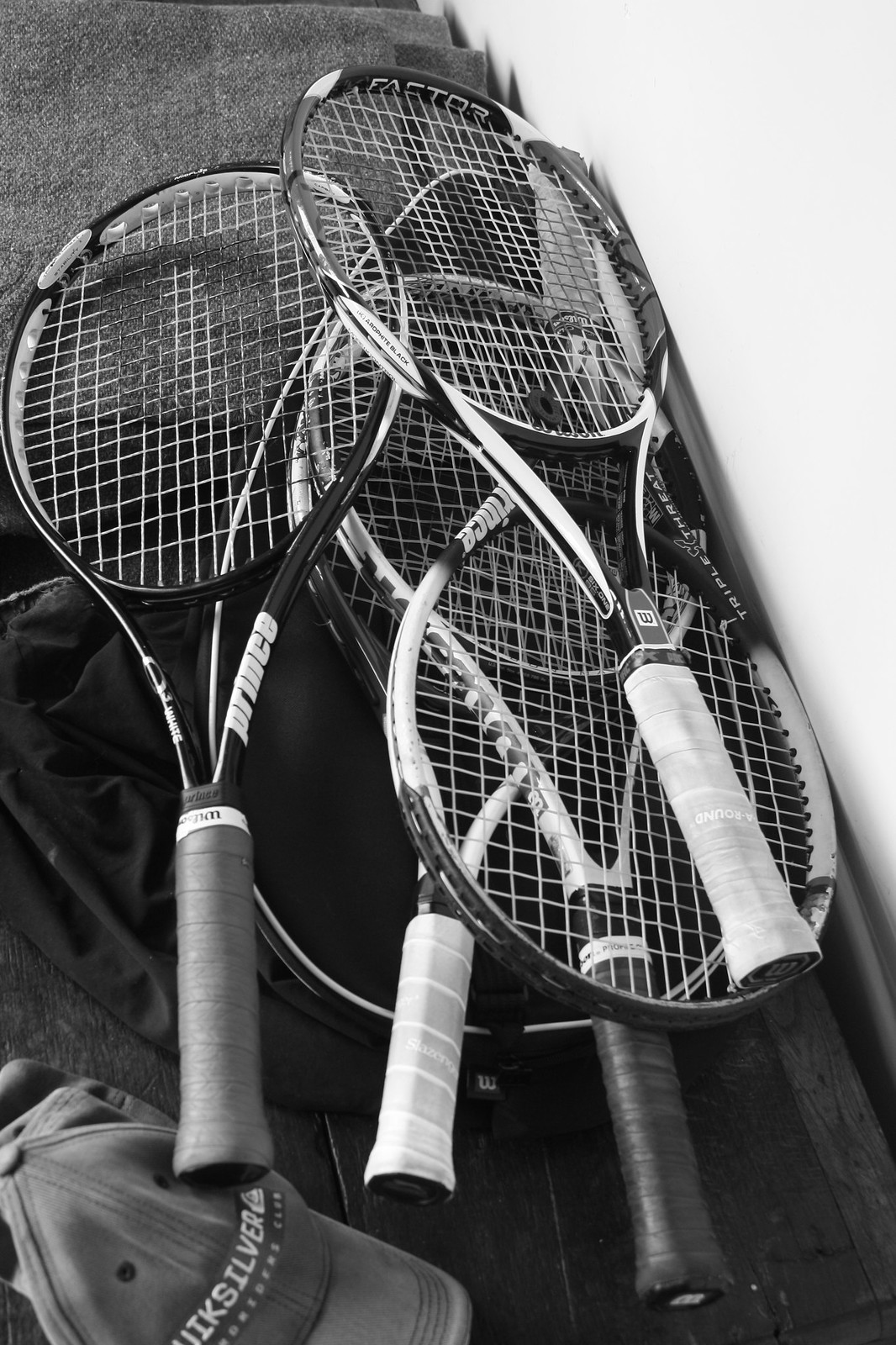A high-resolution black and white digital photograph captures an artistic arrangement of several tennis rackets piled haphazardly on top of each other, with their orientations varied. Most racket handles are pointing towards the viewer, except for one handle pointing away. The rackets, which appear to be of different brands including Wilson and Prince, exhibit distinctly dirtied grips in shades of white, grey, and black, indicating they are well-used. At the bottom left corner of the image, a partially cut-off gray baseball cap with the word "Quicksilver" written on it in white lettering can be seen. The rackets are spilling over a black racket bag onto what seems to be a folded grey cloth or a ruffled blanket. A white wall occupies the right side of the image, stretching from the upper right to about three-quarters down the photo. The light source, coming from the left, casts low shadows of the rackets onto the wall, suggesting it is daytime.